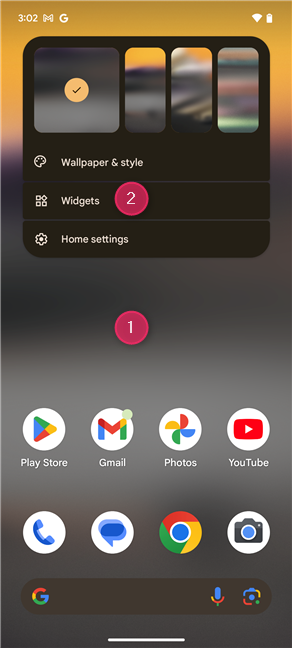In this detailed screenshot of an Android mobile device, we observe a rectangular image that is taller than it is wide.

At the very top left, the status bar displays the time as "3:02", accompanied by three white icons: a "M" icon, a "G" icon, a signal strength icon, and a battery icon. These elements are set against an orange background that seamlessly fades to gray roughly one-fifth down the screen.

Positioned around the transition from orange to gray, there is a prominent black box containing four smaller boxes with various patterns, likely representing wallpaper options for the phone. Beneath this section, we encounter text in white: "Wallpaper & style," followed by "Widgets," highlighted with a pink circle bearing the number "2" inside it. Continuing downwards, the text "Home settings" is present.

Further down the screen, there is a prominent pink circle with the number "1" inside it. Below this, we find a row of commonly used app icons: the Play Store icon (a multicolored triangle), the Gmail icon (a multicolored "M"), the Photos icon (a multicolored pinwheel), and the YouTube icon (a red button with a white play triangle).

The next row features a suite of communication and browsing icons: a phone icon inside a white circle, a message box icon inside a white circle, the Google Chrome icon, and a camera icon inside a white circle.

At the very bottom, there is a comprehensive search bar displaying the Google "G" logo, an expansive blank space meant for text input, and icons for a microphone and a camera, providing quick access to voice search and image search functionalities.